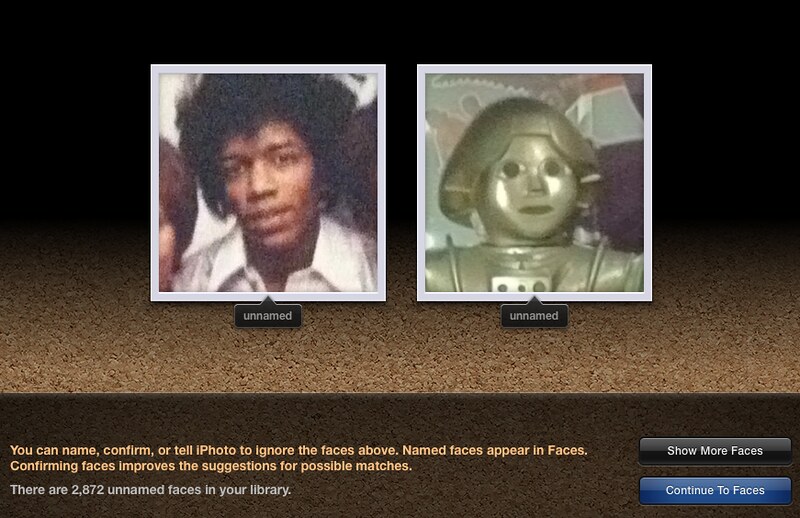The image features two grainy photographs set against a black background that transitions into a brown ombre effect. The first photograph on the left is a close-up of an African-American man with an afro, dressed in a white t-shirt, bordered in silver. The second photograph on the right is of a golden robot, reminiscent of R2D2 or C-3PO, also bordered in silver. Both images have the label "unnamed" beneath them. Below these photos, text reads: "You can name, confirm, or tell iPhoto to ignore the faces above. Named faces appear in Faces. Confirming faces improves the suggestions for possible matches." Additionally, it notes, "There are 2,872 unnamed faces in your library." In the bottom right corner, two buttons are displayed: a black "Show More Faces" button and a blue "Continue to Faces" button. The overall layout and text suggest that this is part of a tutorial or instructive interface for using iPhoto.